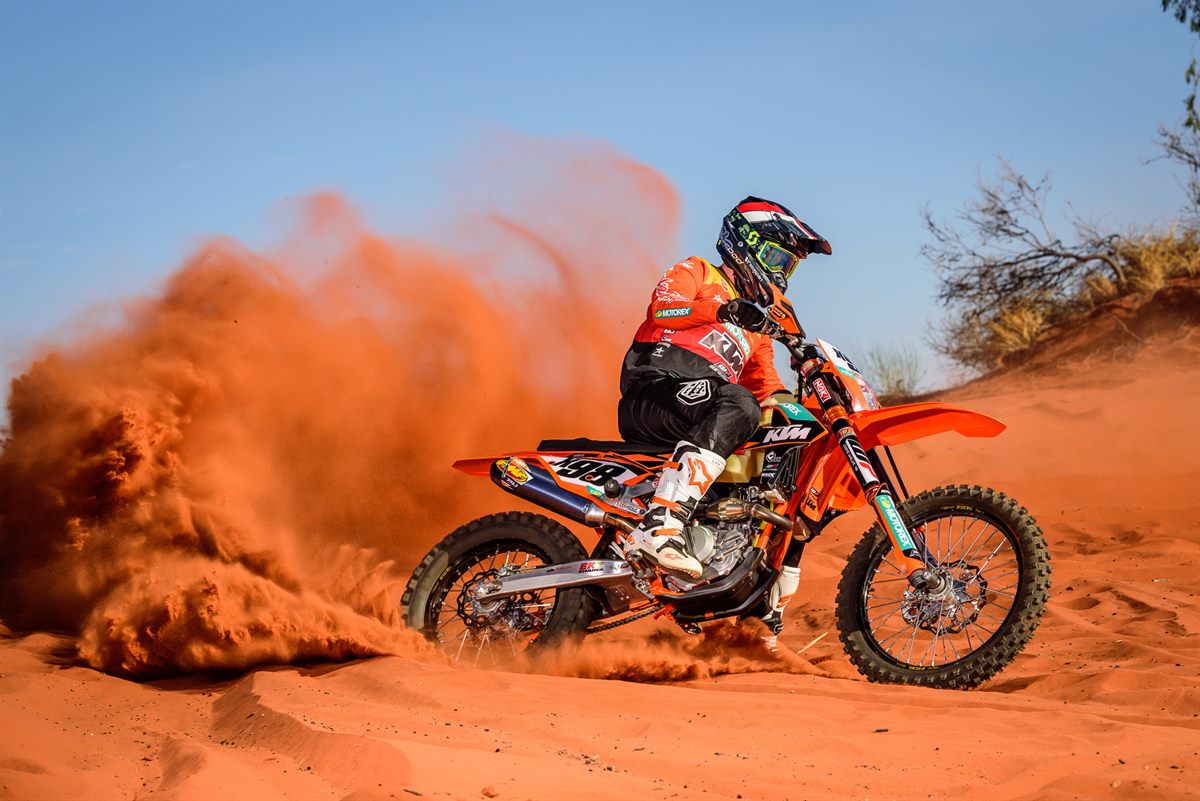In this vibrant photograph, a man on a dirt bike is navigating the desert terrain, kicking up a striking cloud of reddish-orange sand into the air. The scene is set under a clear, brilliant blue sky, devoid of clouds and illuminated by the bright sun, which accentuates the vivid colors. The rider, clad in a dynamic racing kit, sports black pants, white boots with orange and black accents, and a long-sleeved shirt in shades of orange and yellow adorned with various emblems and advertisements. His protective gear includes black gloves, an orange, white, and black helmet, and black and yellow or lime green goggles. The dirt bike itself is predominantly orange with hints of black and white, and a number 98 is visible on it. As he descends a sandy hill, the bike's robust tires grip the clay-colored ground, creating an impressive, swirling trail of displaced sand that captures the essence of speed and adventure.